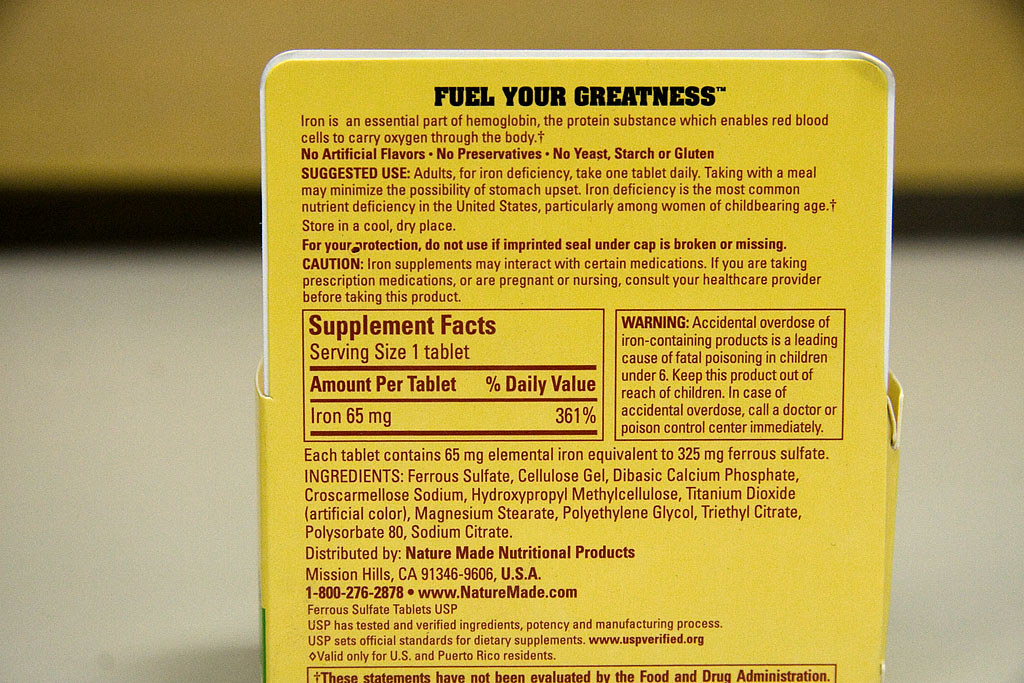A yellow, rectangular package, positioned prominently on a counter, dominates the foreground of the image. The background is artfully blurred, ensuring that the viewer's attention remains on the packaging. Bold black letters at the top of the package declare, "Fuel Your Greatness." Beneath this, smaller, dense red text provides detailed usage directions, cautions, supplemental facts, and warnings, all segmented into neat rectangular areas. The packaging also includes a comprehensive list of ingredients, distributor information, a phone number, and a website, reflecting an emphasis on transparency and consumer information.